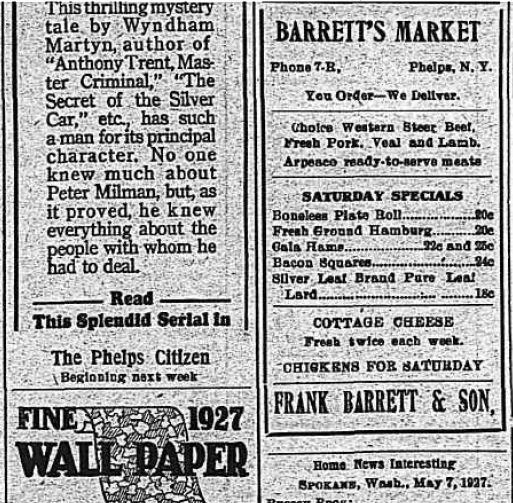This black-and-white image is a scan of an aged, possibly 1927 newspaper sheet, showing a captivating snapshot of its era. On the left side, the text begins with an advertisement for a mystery serial by Wyndham Martin, the author of "Anthony Trent, Master Criminal" and "The Secret of the Silver Car." The partial text reveals the tale's intriguing protagonist, Peter Millman, who secretly knew everything about the people he dealt with. Beneath this, an announcement encourages readers to follow the serial in the "Phelps Citizen," indicating it will begin the following week. Further down, a clearly visible advertisement declares "Fine Wallpaper, 1927."

On the right side, the header "Barrett's Market" stands out, alongside a promotional message: "Phone 7B, Phelps, New York. You order, we deliver." Below this, the 'Saturday Specials' are listed, featuring cottage cheese, freshly stocked twice a week, and chickens available for Saturday. The advertisement is signed by "Frank Barrett and Sons." Scattered black granulated points across the paper, along with its overall weathered appearance, enhance the historic and nostalgic feel of this snippet from the past.